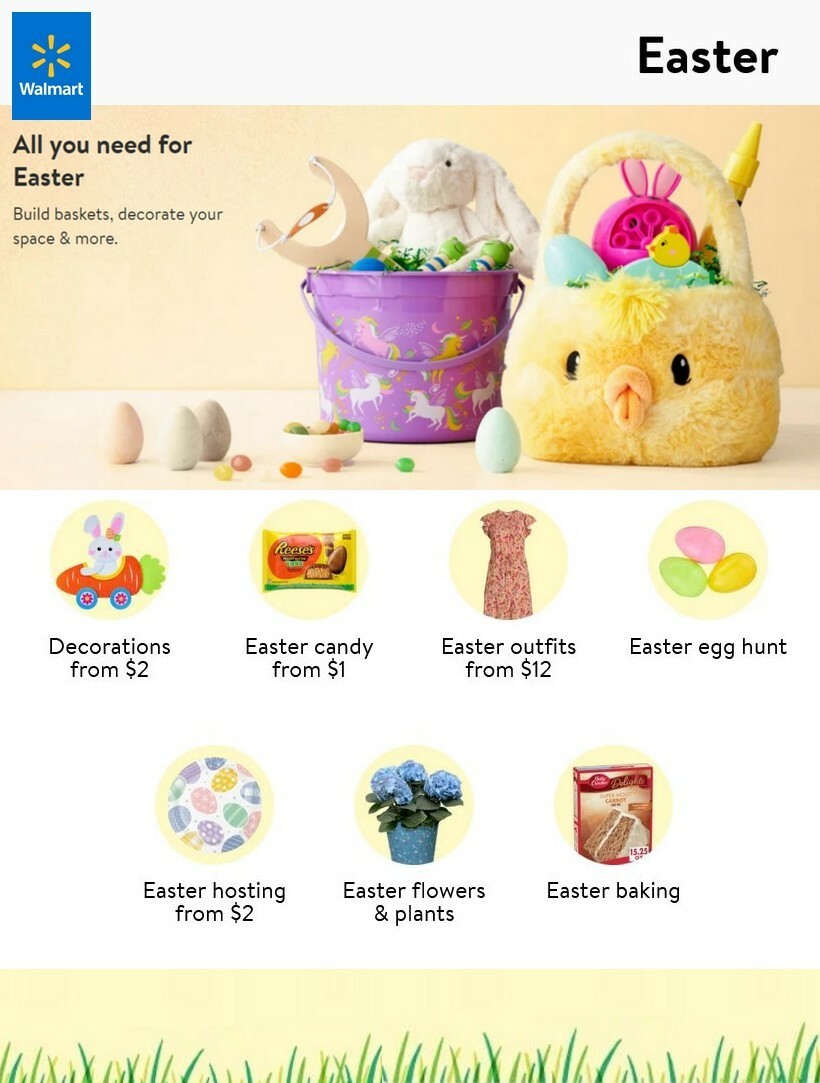This image from Walmart's website features a detailed Easter-themed layout. The top inch and a half of the image is framed with a light gray border. In the top left corner, there is a blue square with the Walmart logo in white. Adjacent to the logo is a sun ray-like symbol composed of six yellow lines. To the right, bolded in black, is the word "Easter."

The main section of the image is set against a tan background. In the top left, bolded text reads, "All you need for Easter." Below this, in smaller black text, it says, "Build baskets, decorate your space." 

In the center of the image, there are several Easter-themed items displayed horizontally:
1. **Three decorated eggs** at varying heights.
2. **A white bowl filled with jelly beans**.
3. **A purple pan** featuring a rabbit, grass, and candy.
4. **A fuzzy yellow purse resembling a bird**, containing Easter toys.

The bottom portion of the image is dominated by a white border with various Easter-themed offers within circular icons, all set against a tan background:
1. **Top left**: A circle featuring a bunny riding a carrot-car icon, with the text "Decorations for $2."
2. **Next**: A circle containing Reese's candy, stating "Easter candy from $1."
3. **Next**: A circle highlighting a red dress with the text "Easter outfits from $12."
4. **Next**: A circle depicting pink, yellow, and green jelly beans, labeled "Easter egg hunt."
5. **Bottom left**: A circle with a plate of various color patterns, stating "Easter hosting from $2."
6. **Next**: A blue flower pot with three blue flowers, labeled "Easter flowers and plants."
7. **Next**: A depiction of a cake mix with the text "Easter baking."

The image concludes with a final inch-wide tan border at the bottom, adorned with small pieces of green grass sprouting upwards.